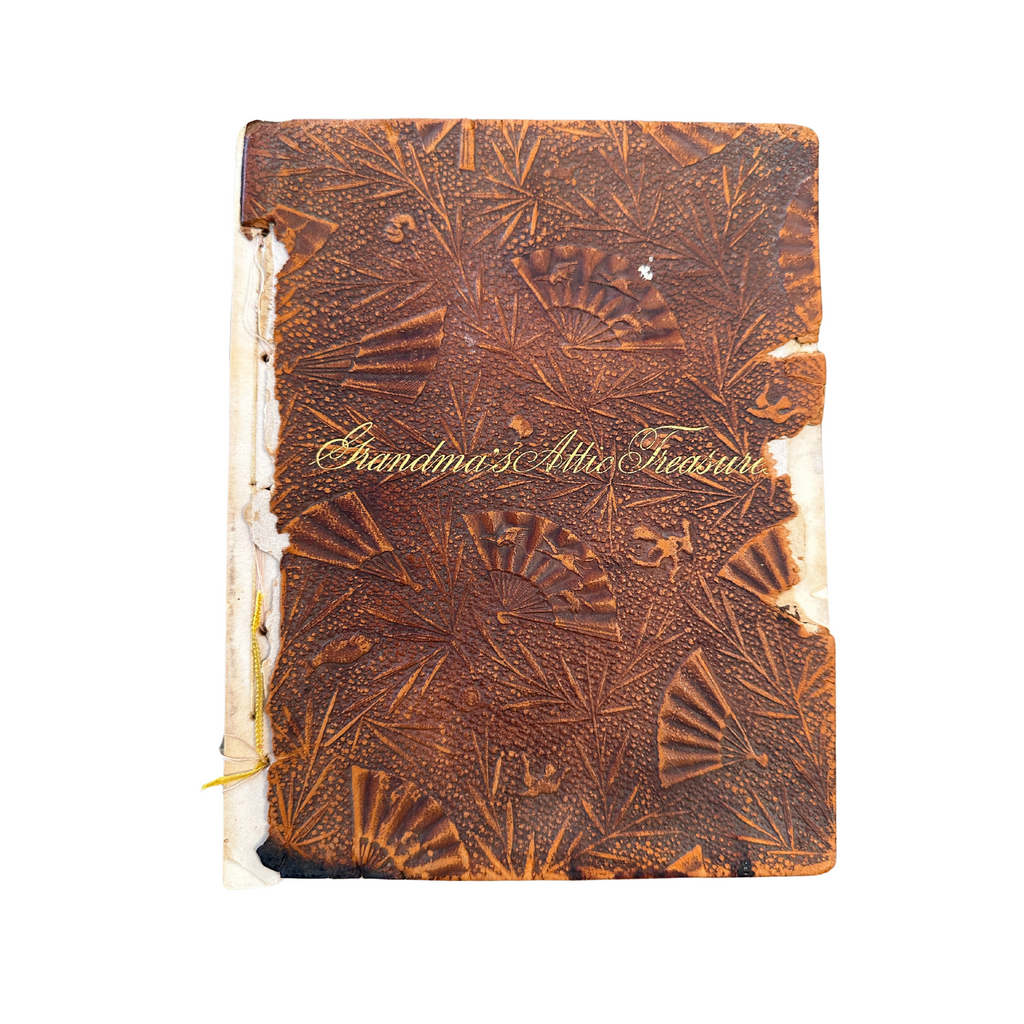This is an image of an old, weathered book titled "Grandma's Attic Treasure" in elegant gold cursive script. The cover, made of tan to dark brown leather or possibly faux leather, is adorned with raised decorations of Chinese hand fans, leaves, and twigs, creating a tactile experience when touched. The book shows significant signs of aging and damage; the spine is partially missing, revealing the white paper and yellow threading beneath the leather. There are additional tears along the edges, particularly on the left side where the book appears to be burnt. The embossed decorations have worn off in some areas, exposing a lighter brown beneath the darker surface. Despite its dilapidated state, the book's title remains intact and prominently displayed.